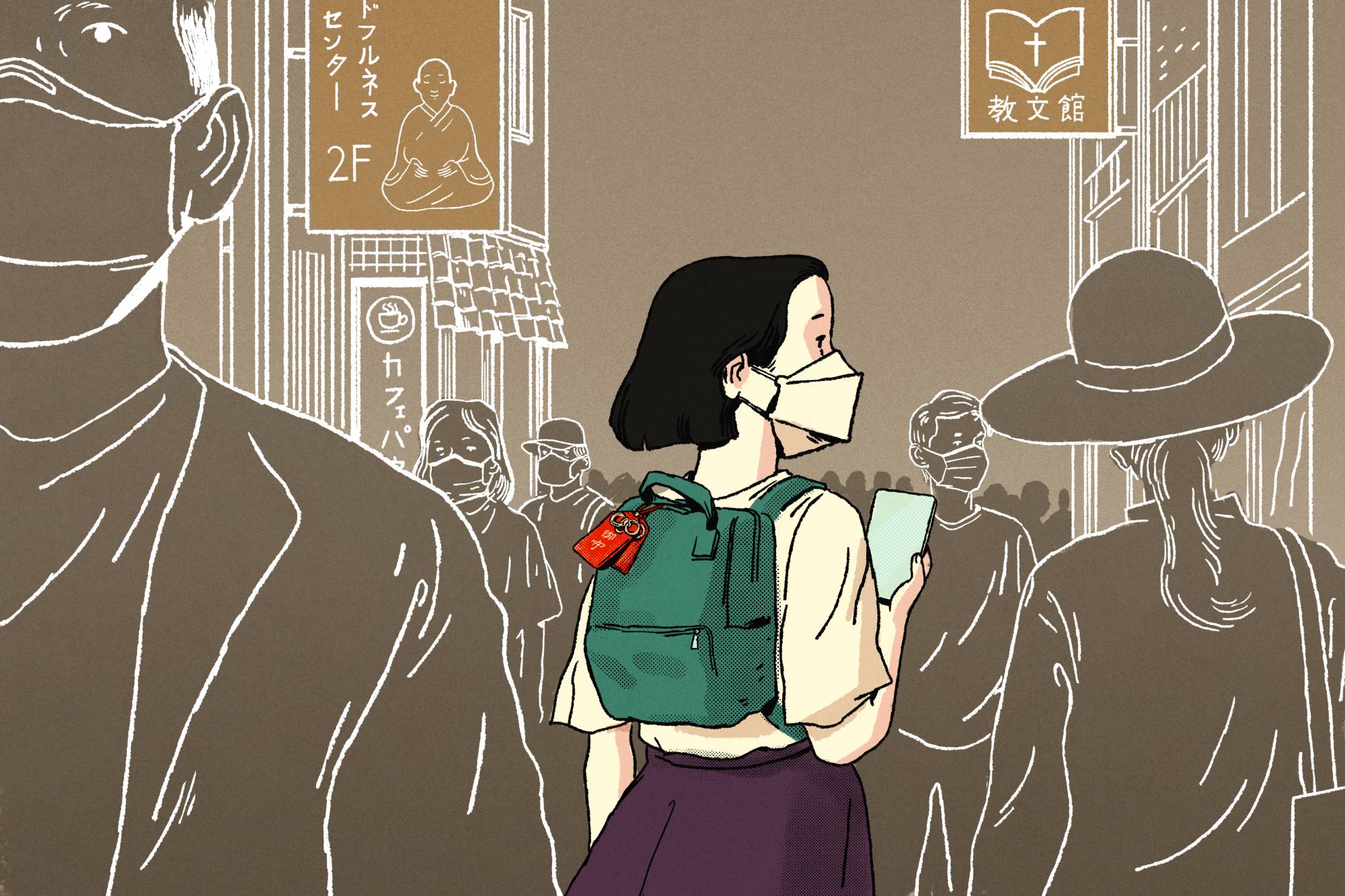The image depicts a detailed illustration, reminiscent of an anime or animated show, set in a bustling street scene of an Asian city, potentially Japanese or Chinese. The focal point is a single young woman who is fully colored, making her stand out against the grayscale background and people. She is depicted with a tan-colored shirt, a purple skirt, and a hunter-green backpack adorned with a couple of red tags. She wears a large tan mask covering her mouth and nose, and her black hair frames her face. In her right hand, she holds up a grayish-white cell phone, glancing off to the side. 

The scene is filled with numerous people walking around, all illustrated as monochromatic or brown figures with white detail lines, and they all wear masks. The woman in the foreground stands out as she walks down the center of the alleyway. To her right, a woman with a large, wide-brimmed hat is noticeable. The street is flanked by buildings with distinct signage: one side features a church with a sign displaying a cross on a book, indicative of a Bible, while the other side has what appears to be a Buddhist temple with a monk meditating cross-legged. Above her and to the left, additional signs in honey-colored brown with numbers and Chinese symbols are visible.